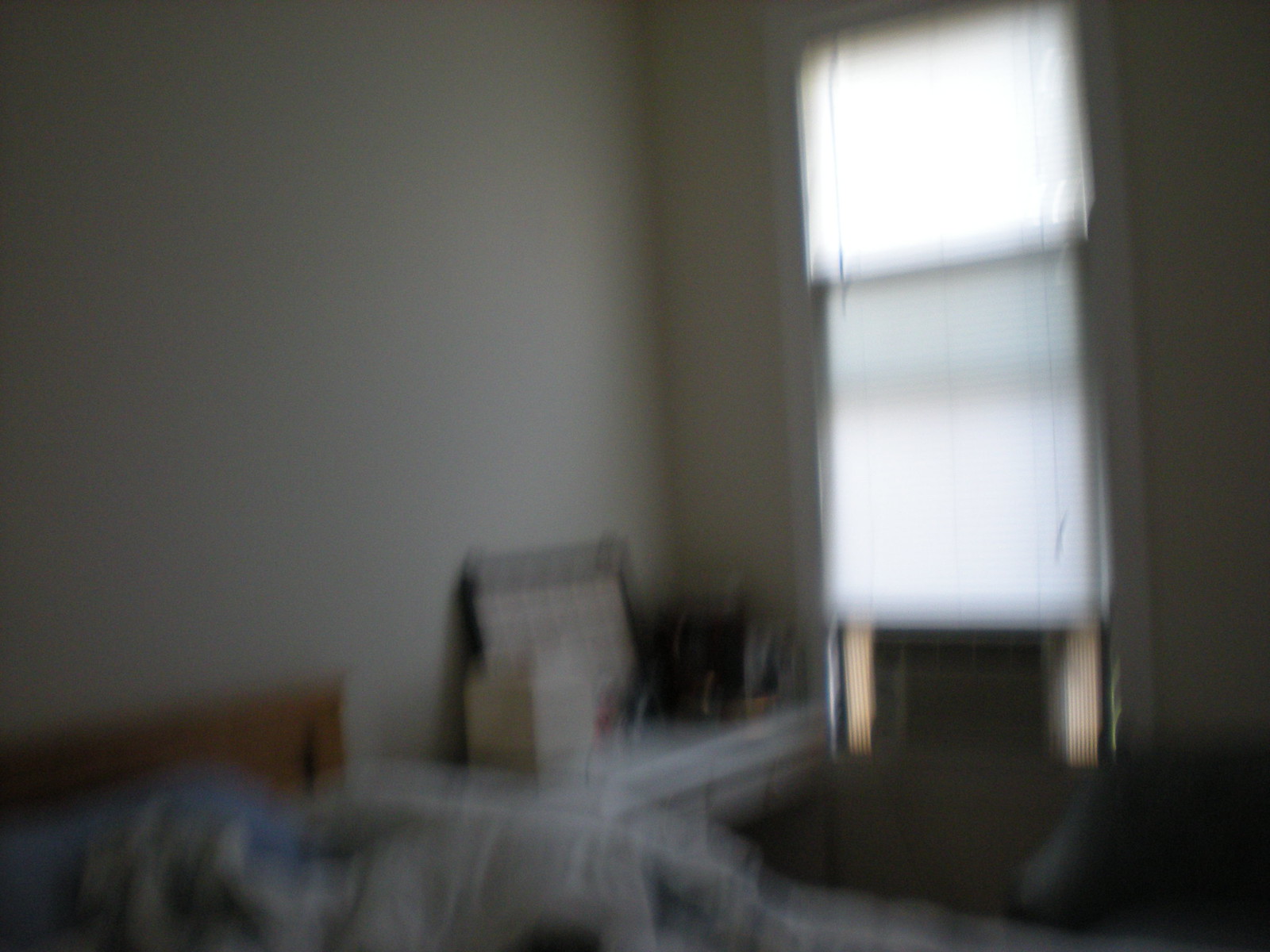In this blurry image of a bedroom, the bottom left-hand corner features a bed with a light wood headboard. The bedspread is disheveled, indicating a jumble of a comforter. To the right of the bed sits a dresser, complete with a mirror and assorted items resting on its surface, though the finer details are indistinguishable due to the blur. On the right-hand side wall, a closed window with blinds filters light into the room. The window is also fitted with an air conditioner unit, with the device's sides extending outward to secure it in place.